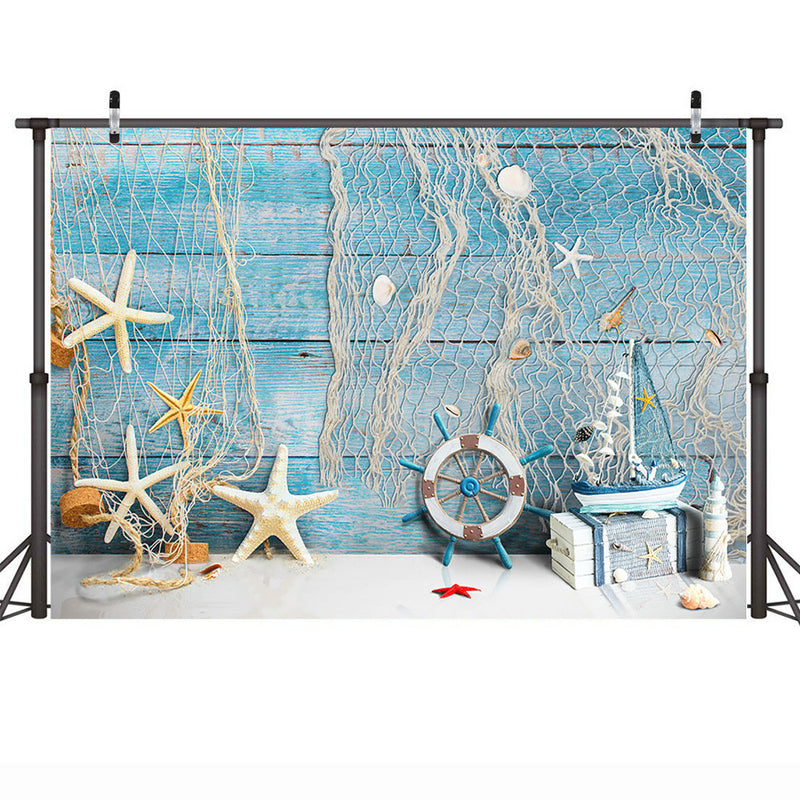The image depicts a nautical-themed indoor scene set against a backdrop of horizontally laid blue-painted wooden panels. A tan fishing net is draped artistically over these panels, adorned with various maritime items. To the left side of the net, there are several starfish ornaments, predominantly white or off-white, with one starfish appearing in shades of yellow and orange, all showcasing the typical five-legged starfish design. The lower center and right portions of the net feature a prominent ship's wheel, painted white with brown squares marking the cardinal points, and blue handles used for steering. Additional nautical decorations include a small wooden chest and a miniature boat positioned just above it, along with an ornamental lighthouse. The entire setup is clipped to a gray metal frame, visible at the top and sides of the image, lending an organized display quality to the scene. The backdrop extends to a white base, against which the decorative elements are arrayed, creating an evocative seaside ambiance.